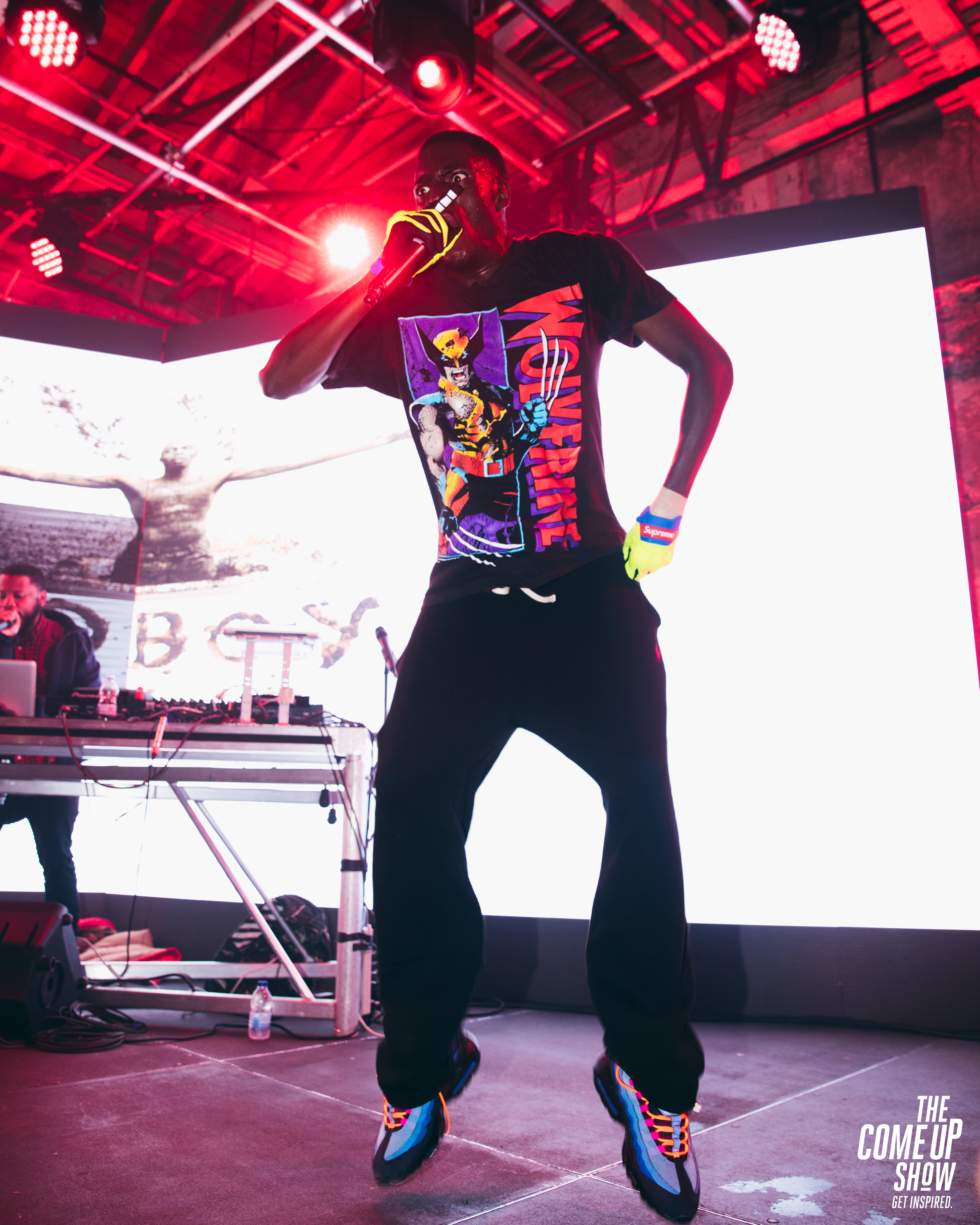The photograph captures a dynamic moment of a man performing on stage in an indoor venue, evidenced by the visible roof with various metal support pipes, scaffolding, and multiple LED spotlights. The man appears to be in mid-jump, lending a sense of energy and animation to the scene. He is dressed in black pants and gray shoes featuring a blue stripe and black bottoms. He wears a black graphic t-shirt showcasing a cartoon image of the comic book character Wolverine, with the name "Wolverine" in orange lettering on the front. His attire is completed with yellow and dark biking gloves. The concrete, squared, tiled floor displays wet spots, enhancing the realism of the setting. The man holds a microphone in his right hand while his left hand rests on his hip, and his gaze is directed towards the left side of the frame. In the background, a DJ setup, including a computer, is visible alongside a screen projecting a display. At the bottom right of the image, white text reads: "The Come Up Show Get Inspired."